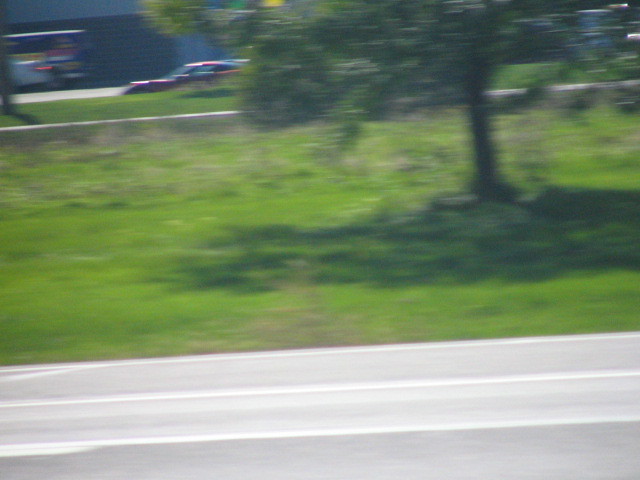The image depicts a scene viewed from a speeding vehicle, likely shot out of a side window. The foreground features a light gray road with several horizontal white stripes. Adjacent to the road, there is a grassy median characterized by light green grass with sporadic darker brown patches, indicating dead spots. A large tree with a dark, indistinct trunk and full green leaves stands prominently in the middle-right of the frame. In the background, beyond another strip of road, is a red car located in the top left corner. Behind the red car, there appears to be another vehicle, possibly a multicolored van or truck, parked alongside a building. The image is slightly blurred, emphasizing the motion of the vehicle from which it was taken. The lighting suggests it was taken during the day, as indicated by the sunlight glare and the shadows around the tree.